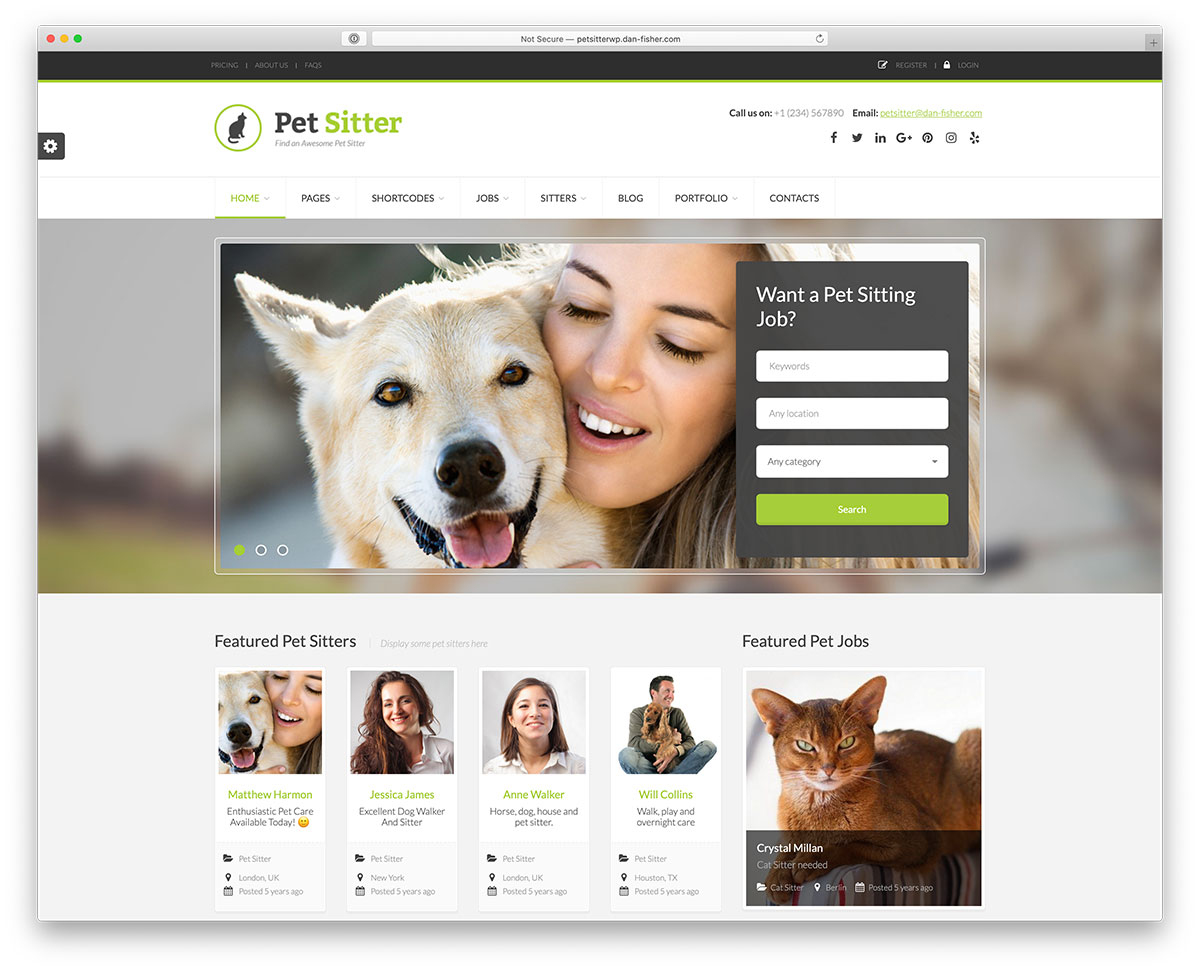The image is a detailed screenshot from a computer displaying a webpage from the website "PetSitter." The website's name is prominently positioned in the top left corner, accompanied by an image of a cat. On the right side of the header, there is contact information along with icons for various social media platforms, though the contact details are somewhat small and difficult to discern.

Below the header, the navigation menu includes options for Home, Pages, Shortcodes, Jobs, Sitters, Blog, Portfolio, and Contacts. 

The main content features a central image of a woman affectionately pressing her face against a tan and white dog. She is smiling with her eyes slightly closed, conveying a moment of tenderness and joy. This image is superimposed on a blurred background, which adds a soft focus to the scene.

To the right of the woman's head, there's a text box that reads, "Want a Pet Sitting Job?" Below this prompt, there are input boxes for keywords, a secondary entry that is unclear, a dropdown menu labeled "Any Category," and a prominent green search button.

At the bottom of the page, there's a section titled "Featured Pet Sitters," showcasing four different profiles. To the left, a separate section labeled "Featured Pet Jobs" includes a picture of a cat, highlighting available pet sitting positions.